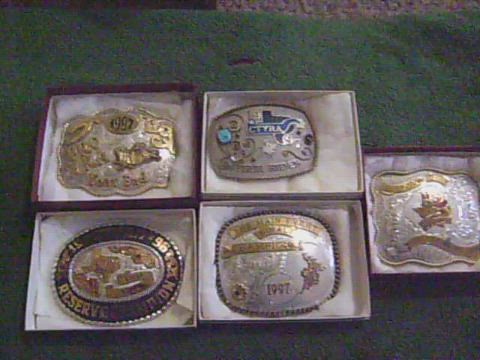This color photograph displays five boxes arranged on an artificial green grass surface. Four boxes are positioned in a square formation, with two rows of two, and a fifth box is placed to the right of this formation. Each box contains a belt buckle, nestled in white cushions. The belt buckles have various designs and inscriptions. The top left buckle is a combination of silver and gold, with "1997" inscribed at the top and an emblem resembling Texas in the center. The buckle on the top right is square-shaped with silver and blue designs, including a noticeable chunk of turquoise at the top left corner. The bottom left buckle is round with a black border and gold writing, featuring a white and gold interior and an image of Texas. The bottom right buckle, also square, is silver with gold inscriptions and "1997" marked at the bottom. The lone box to the right holds another square buckle, characterized by gold writing against a silver background.